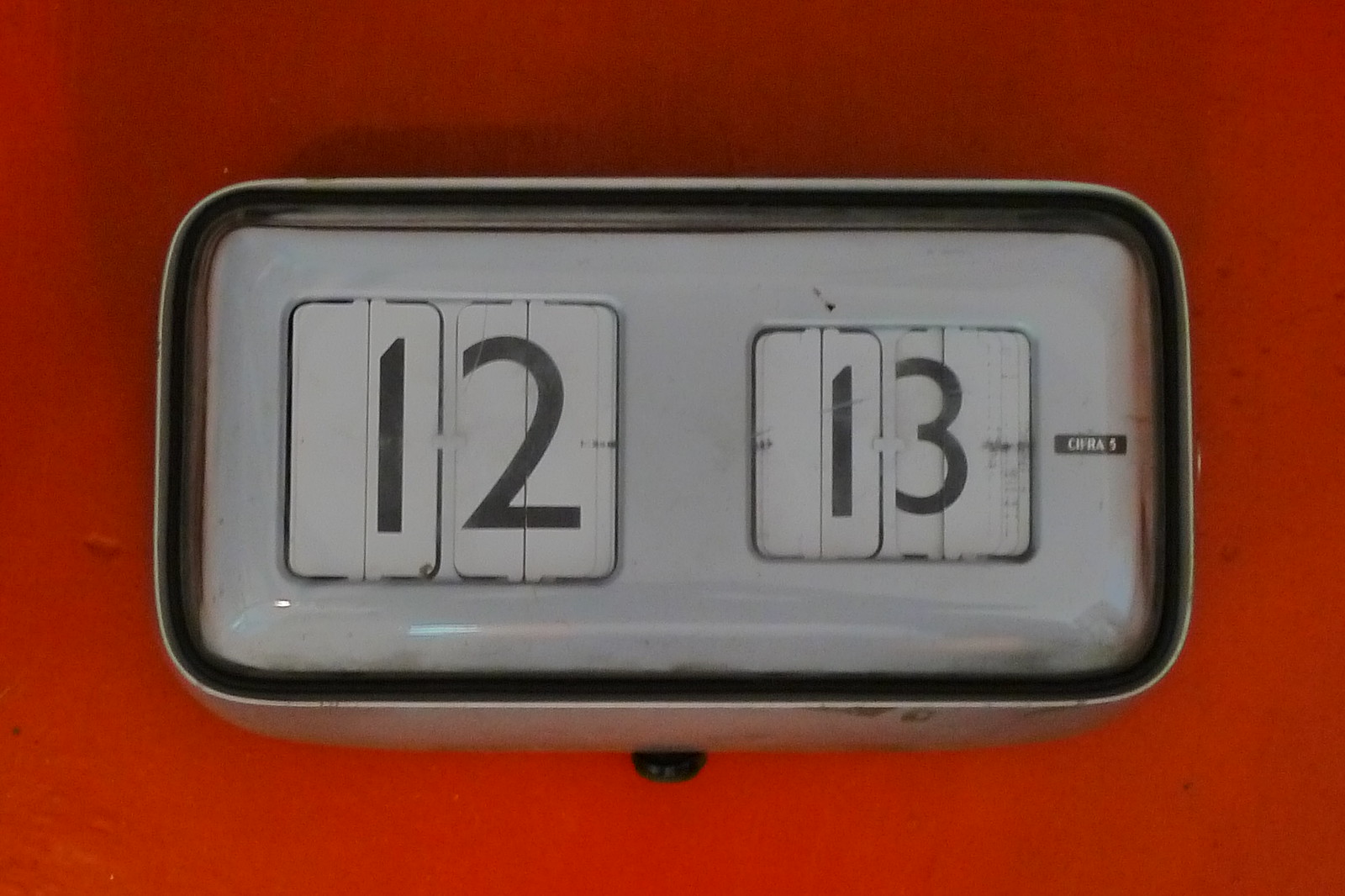The image showcases a vintage, rectangular clock with white metal casing and a clear, intact glass front. The clock, viewed from above, features a white face displaying numbers 12 and 13 in black, using a mechanical flip mechanism. A small rectangular box to the right of the numbers has indistinguishable text. There is a small, black round dial at the bottom likely for setting the time. The clock rests on a surface with a dark reddish-orange background, possibly a table or nightstand. The letters "CWRA5" appear near the display. The overall scene is taken in real color, emphasizing the clock's classic, old-fashioned design.